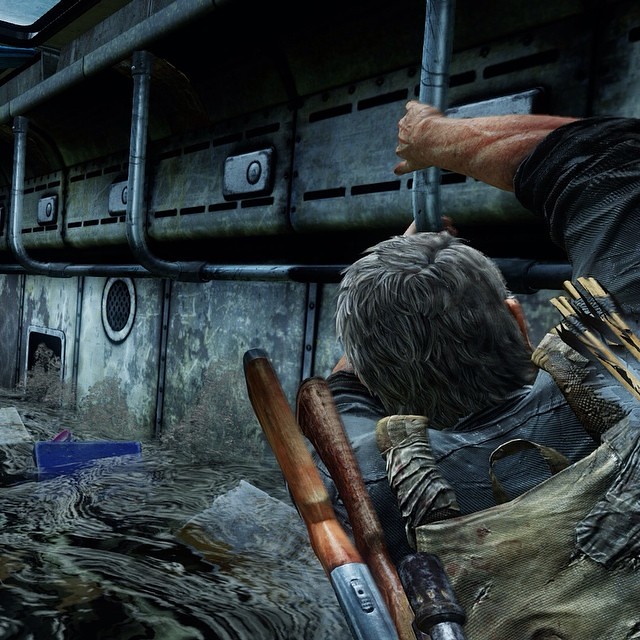The image portrays a highly detailed, possibly digital drawing of an interior scene with metal walls, giving the space an industrial feel. The overall color scheme is dominated by dark gray tones, highlighted by ambient lighting that creates a moody atmosphere. 

At the top of the composition, metal shelving and a network of pipes are visible. These pipes extend downward before disappearing back into the wall, contributing to the mechanical complexity of the setting.

In the bottom left corner, the floor of the space is partially submerged in water, suggesting either a malfunction or a flooded area. A distinct blue object, resembling a floating rectangle, is partially visible just above the waterline.

The focal point of the image is the back of a man positioned prominently on the left side. His hair is a mix of salt and pepper, indicating age or stress. His right arm is extended upwards, clutching a pipe attached to the ceiling. He is dressed in a dark long-sleeve shirt, the sleeve pushed up to reveal his forearm. The man is also wearing a backpack, from which the handles of tools or possibly weapons protrude, extending from both the left and right sides, hinting at his preparedness or profession.